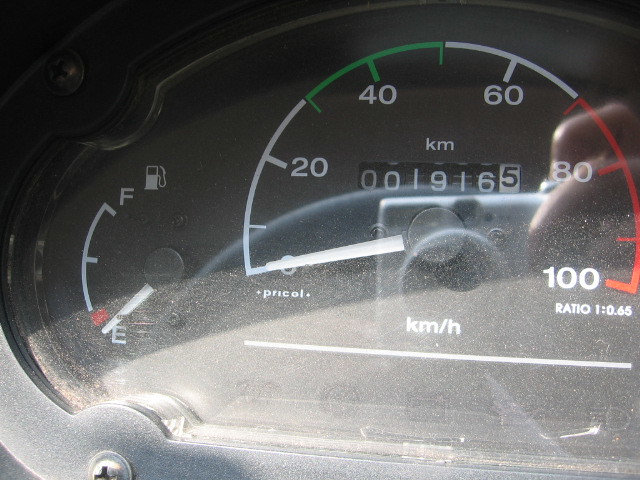This image captures the dashboard of a car, focusing on various crucial instruments. The primary elements include the fuel gauge, speedometer, and odometer, all set against a black background. 

The fuel gauge is distinctly marked with a red line for 'Empty' and an 'F' indicating 'Full.' A small icon resembling a gas pump confirms its function. The gauge itself has a black divot with a white needle currently pointing to 'E,' suggesting that the fuel level is at empty.

The speedometer, centrally located, ranges from 0 to 100. The markings are color-coded: white from 0 to 25, green from 25 to 45, white again from 45 to 65, and red from 75 to 100, indicating different speed intervals. The speedometer needle rests at zero, implying that the car is stationary. The odometer, located at the center of the speedometer, displays a reading of 1,016.5 kilometers traveled.

Notably, a Phillips screw is visible within the circular arrangement of the dashboard instruments, adding a subtle detail to the overall layout. The combination of these elements forms a detailed and informative view of the car's dashboard.